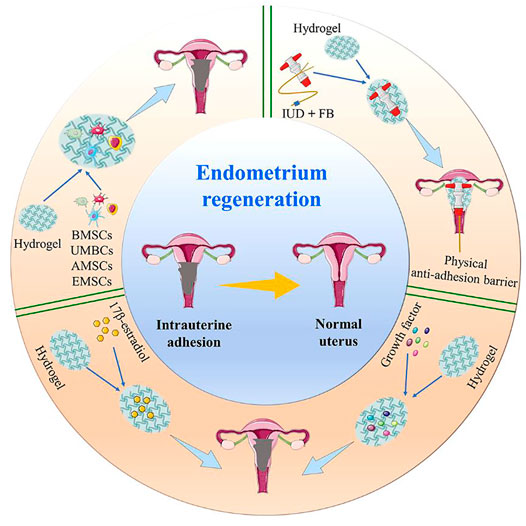This educational graphic features a circular layout against a whitish background, resembling a life raft. The centerpiece is a blue circle labeled 'Endometrium Regeneration,' displaying two diagrams of the uterus and fallopian tubes. The left diagram indicates 'Intrauterine Adhesion,' and the right, labeled 'Normal Uterus,' is connected by a yellow arrow pointing to the right.

Encircling the central blue area is a beige ring marked with various detailed illustrations and labels, beginning at the top (12 o'clock position) and moving clockwise. At the top, it mentions 'Hydrogel, IUD plus FB' alongside a depiction of an IUD, connected by arrows to a uterus, signaling its role as a 'Physical Anti-Adhesion Barrier.' Continuing clockwise, the labels include 'Growth Factor' and 'Hydrogel,' each associated with arrows pointing toward a uterus, indicating their function in promoting endometrial regeneration. The illustrations in the beige ring feature medical instruments and arrows, further explaining the process visually.